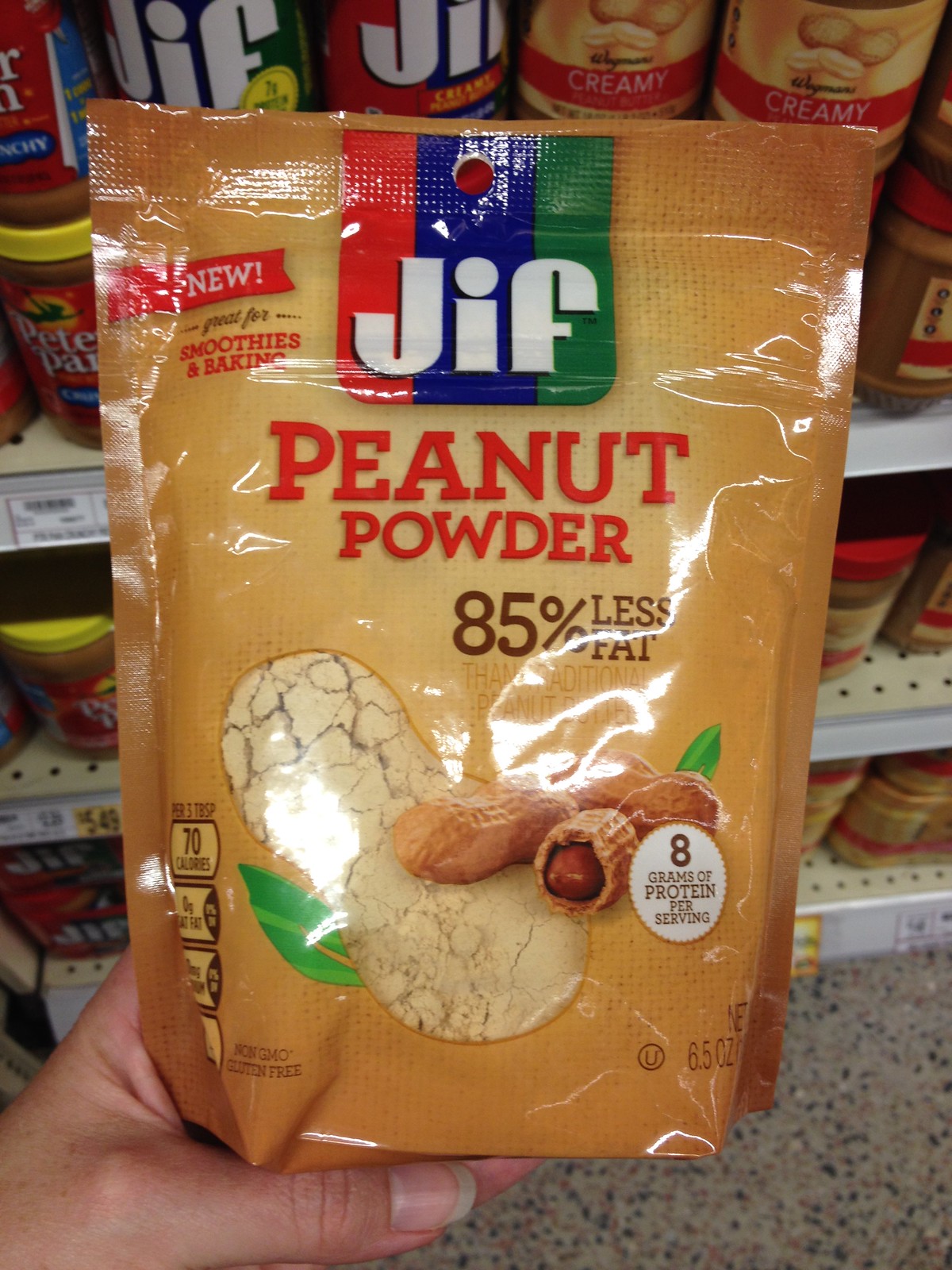In a grocery store aisle, a close-up first-person perspective image captures a packet of food held in a woman's left hand, revealed by her untrimmed thumbnail. The brown packet prominently features a red, blue, and green striped logo at the top with the trademark "GIF" in white. Below the logo, bold red letters declare “Peanut Powder,” followed by “80% Less Fat” in green. Due to a light reflection, some text is partially obscured, but “Peanut Butter” is visible. A graphic of scattered peanuts is accompanied by a white circle stating “8 grams of protein per serving.” Adjacent to the peanut image, a clear window reveals the peanut powder inside. 
Behind the packet, three shelves display various products, seemingly different spreads or peanut butter varieties in plastic jars with screw-on lids. The bottom edge of the image shows a portion of the grocery store floor, characterized by a grey base with black, brown, and purplish spots, likely a marble surface.